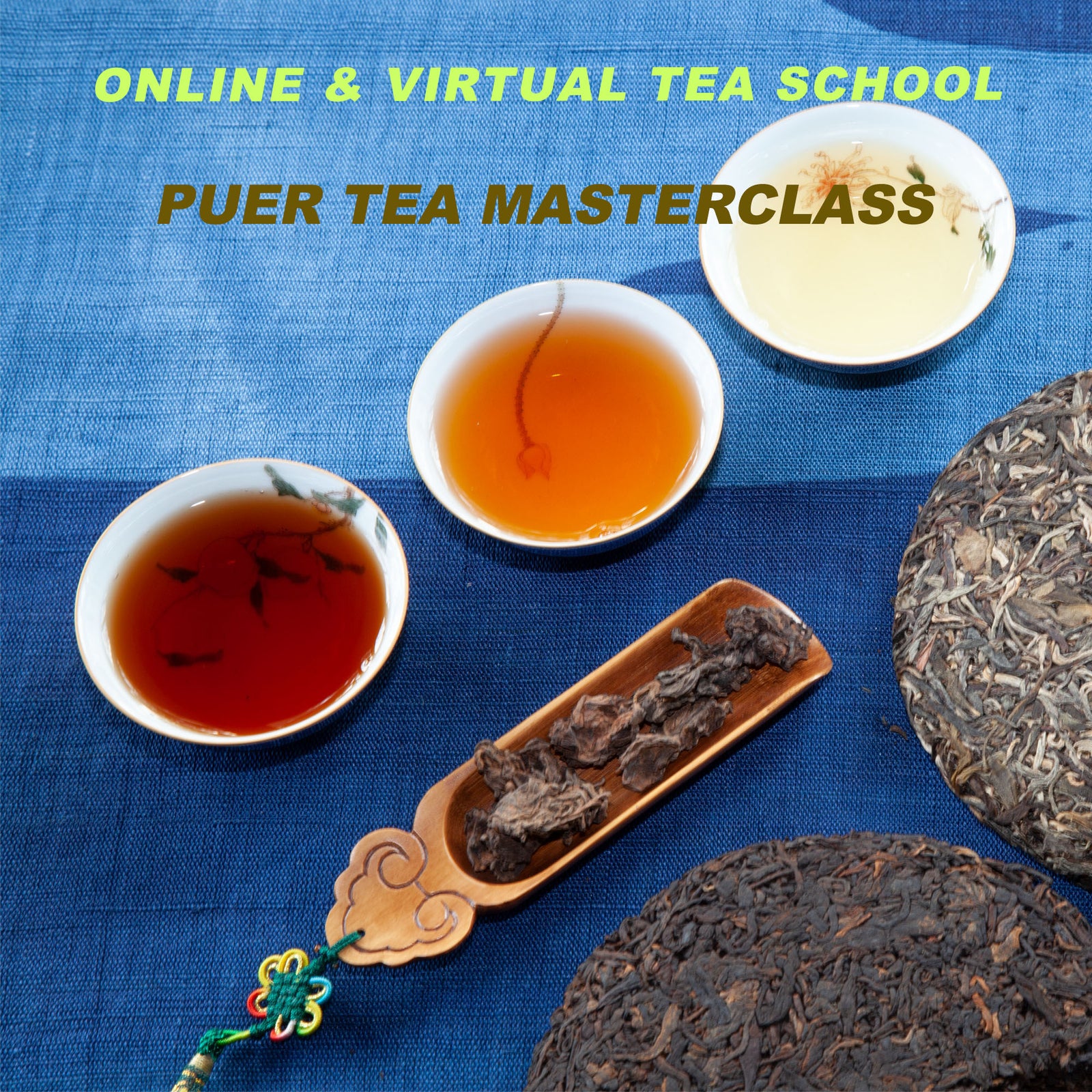This square advertisement image features a vibrant tabletop setting promoting an "Online and Virtual Tea School" with bold, lime-green text. Beneath it, in prominent brown text, the caption reads "Puerh Tea Masterclass." The blue tablecloth on the table has two distinct shades: light blue at the top and navy blue on the bottom. Arranged diagonally across the cloth are three white, circular bowls, each containing a different liquid. The bowls hold a spectrum of teas: the lowest bowl contains a medium-brown liquid, the middle one has an orange liquid, and the top bowl holds a beige liquid. A rectangular wooden incense holder, possibly also a tea tool, sits nearby filled with blackish-gray tea leaves. Additionally, in the bottom right corner of the image, there are compacted circular discs of tea leaves, known as tea bricks. The detailed composition and rich colors create an inviting and informative visual promoting the tea masterclass.